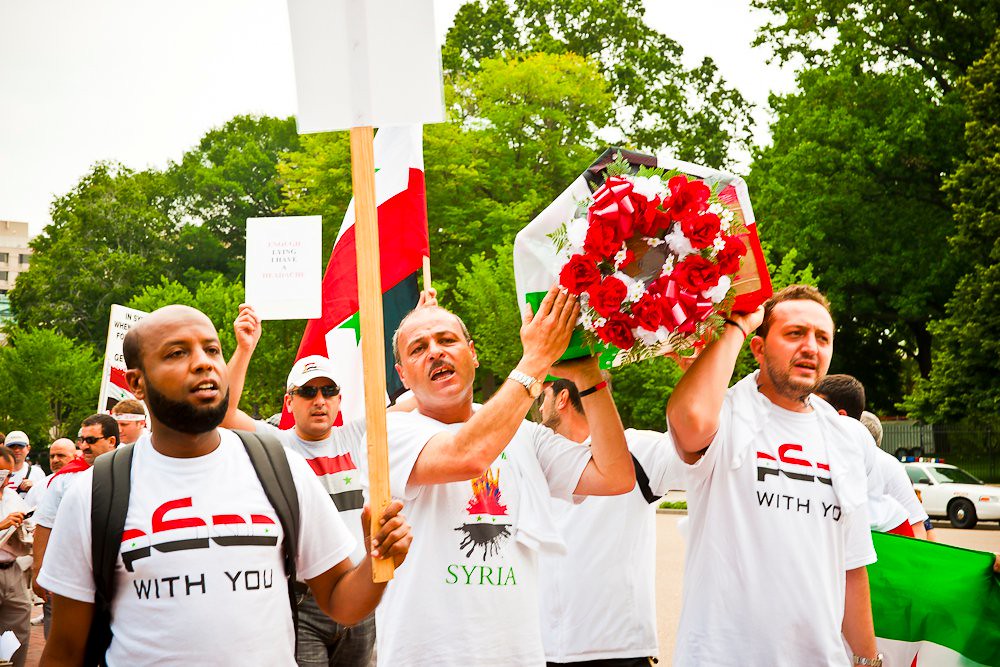This photograph captures a poignant moment at a protest or rally set against an urban backdrop featuring a cityscape and a park brimming with trees and greenery. In the immediate foreground, three men walk with a sense of purpose. The man on the left is clearly visible; he's bald with a beard and wearing a white t-shirt displaying a message partially readable as "with you" along with a red, white, and blue logo. He holds a white poster on a long stick. 

Center stage is an older, middle-aged man, clad in a similar t-shirt but with a distinctive 'Syria' graphic, who holds a small casket adorned with a circle of red flowers. Assisting him on the far right is another man in an identical t-shirt, also supporting the miniature casket hoisted above their heads. 

The scene is set outdoors, with a police car parked by the side of a road that borders the rally area. The trees, flags, and distant buildings frame the scene, creating a vivid contrast of greenery and urban elements. Signs and t-shirts worn by several men in the crowd reiterate solidarity with Syria, with common slogans like "with you Syria." The atmosphere speaks to a collective moment of remembrance or protest, underscored by shared symbols of red, white, and green.